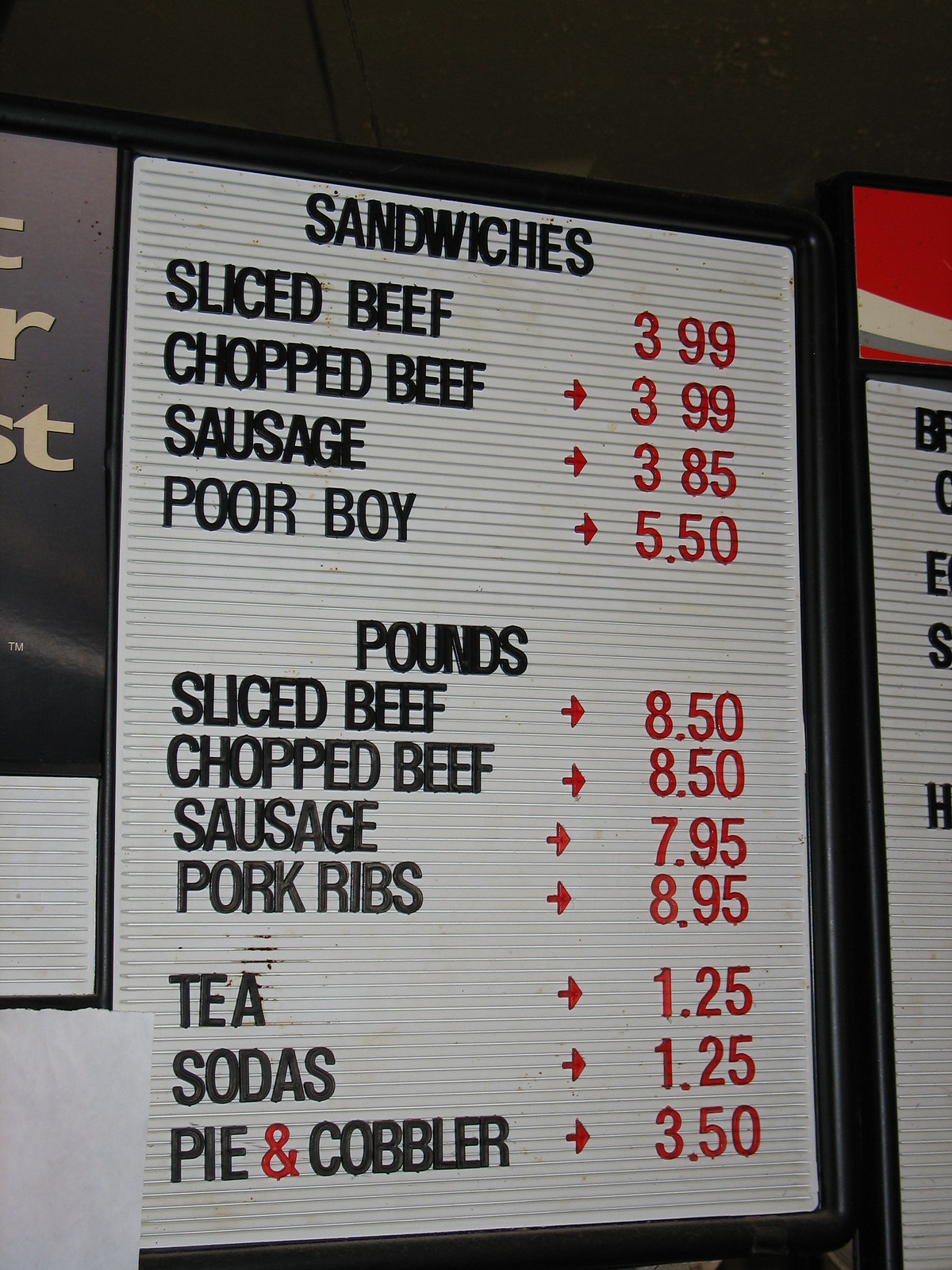This is a photograph of a menu featuring a variety of meal options and their prices. The menu is organized into two columns. On the left-hand side, it lists different types of sandwiches and meats available by the pound: "Sandwiches: Sliced Beef, Chopped Beef, Sausage, Poor Boy" and "By the Pound: Sliced Beef, Chopped Beef, Sausage, Pork Ribs." Beneath these options, it also lists beverages and desserts: "Tea, Sodas, Pie, Cobbler." All item descriptions are primarily written in black text. On the right-hand side of the menu, corresponding prices are displayed: "Sandwiches: $3.99, $3.99, $3.85, $5.50" and "By the Pound: $5.50."